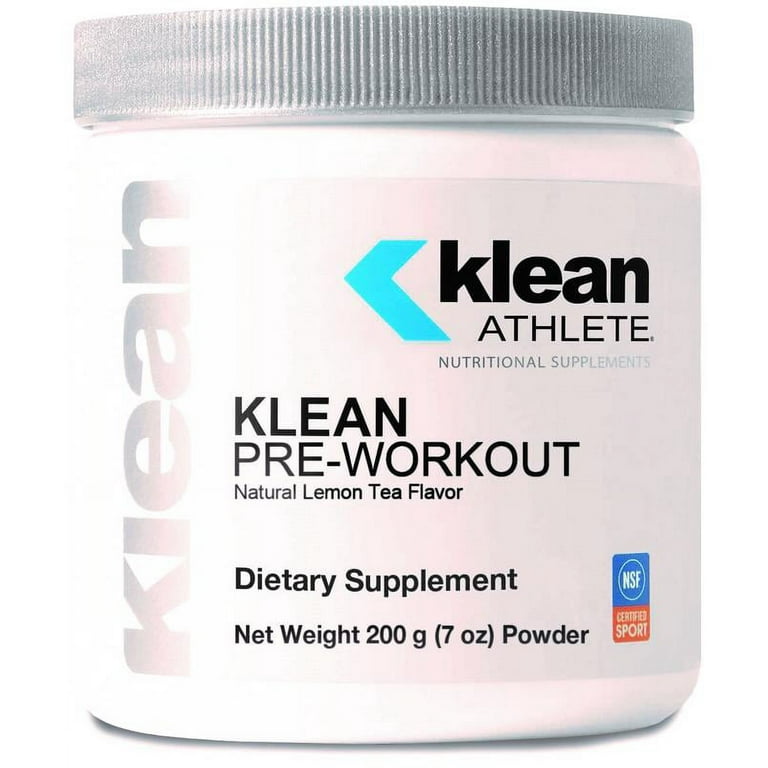This image features a squatty, white, plastic canister approximately four to five inches tall. It has a grayish-silver lid adorned with tiny vertical ridges for grip. The jar prominently displays the brand name "Clean Athlete" with the word CLEAN spelled as K-L-E-A-N in vertically aligned, gray and black text on either side of the canister, accompanied by a teal chevron accent. Below this, in smaller, uppercase letters, the phrase "ATHLETE" is present, followed by "NUTRITIONAL SUPPLEMENTS" in even finer print. At the center of the label, the product is identified as "CLEAN PRE-WORKOUT NATURAL LEMON TEA FLAVOR." The label also mentions that it is a dietary supplement with a net weight of 200 grams (7 ounces). Notably, the label includes certifications such as NSF Certified for Sport but lacks information about the place of manufacture or usage instructions, which might be found on the back of the jar.